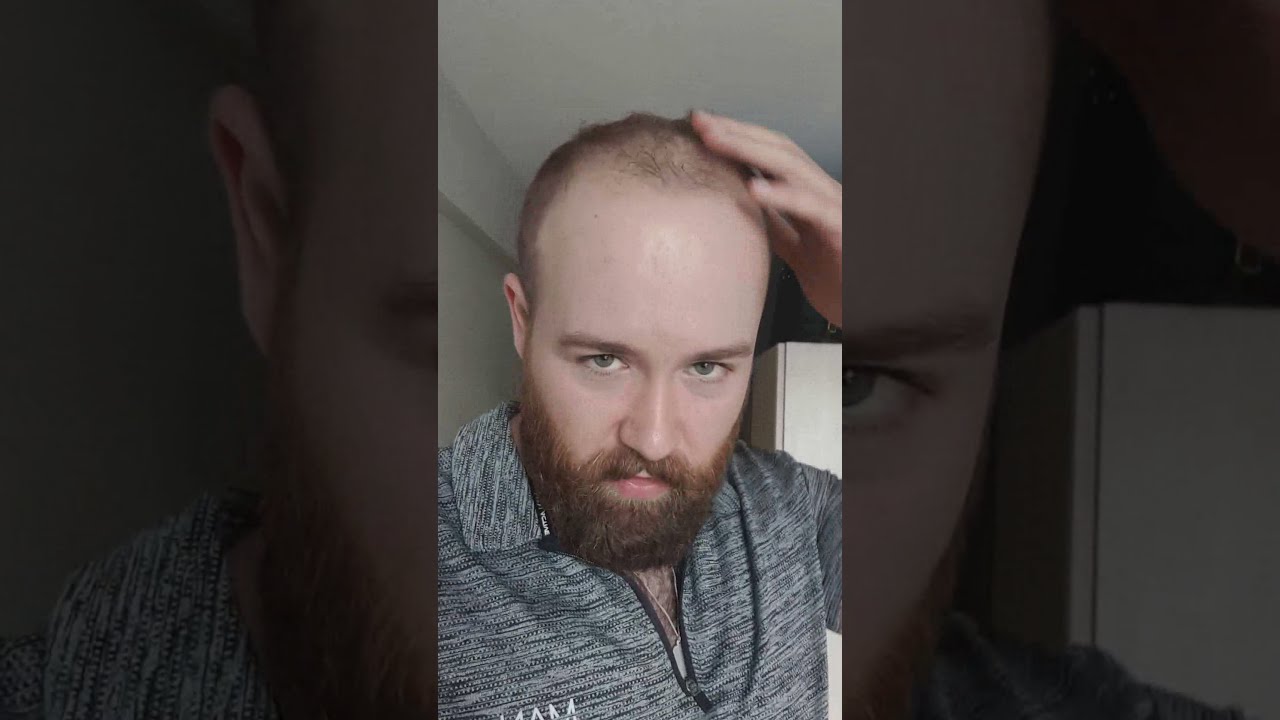This image is a selfie of a man taken in portrait mode on a mobile phone. The man, who is slightly balding, touches his hair lightly with one hand while looking directly into the camera with a dissatisfied expression. He has a receding hairline with sparse hair on top and a contrasting full, thick reddish-brown beard and mustache. His eyes appear to be hazel or blue. He is dressed in a gray long sleeve shirt with a collar and a zipper, displaying a logo on the right side of the chest, and seems to be wearing a dog tag around his neck. The background hints at a room setting with a refrigerator and light-colored walls, possibly indicating a kitchen. Additionally, the sides of the image show a zoomed-in version of his face with a light gray tint, creating a mirrored effect to frame the central portrait.